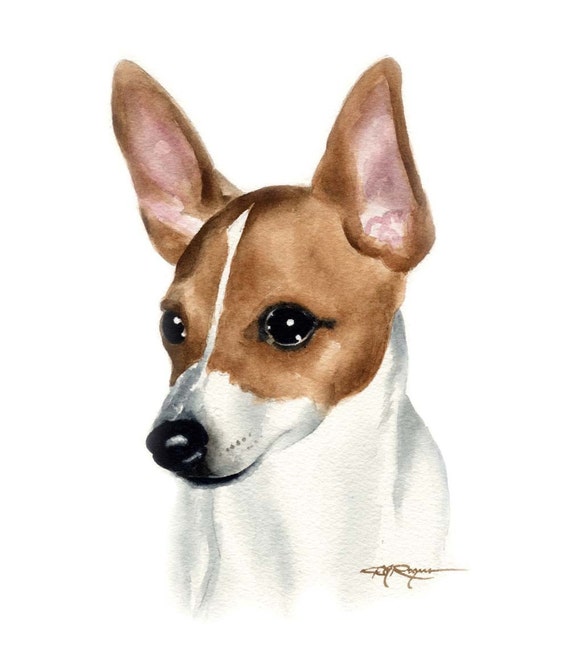This detailed illustration captures a small dog's face with distinctive pointy ears, set against a white background. The dog features a light brown face with angular, smooth-looking fur. A soft pink hue fills the insides of its ears, edged with brown. Notably, a white stripe runs from the dog's forehead down to its muzzle, bisecting its face and enhancing its symmetrical appearance. The muzzle is predominantly white, complemented by a black nose and hints of black around the mouth. The eyes are black, and the dog appears to be looking to the side. The visible portion of the dog's neck and upper body are depicted in an off-white color, adding texture to the illustration. The entire piece resembles a watercolor effect, suggesting the possibility of digital enhancement to emphasize its details. In the lower right-hand corner, there is an artist's signature in brown, though it's illegible and potentially reads Rodriguez or Rogans.